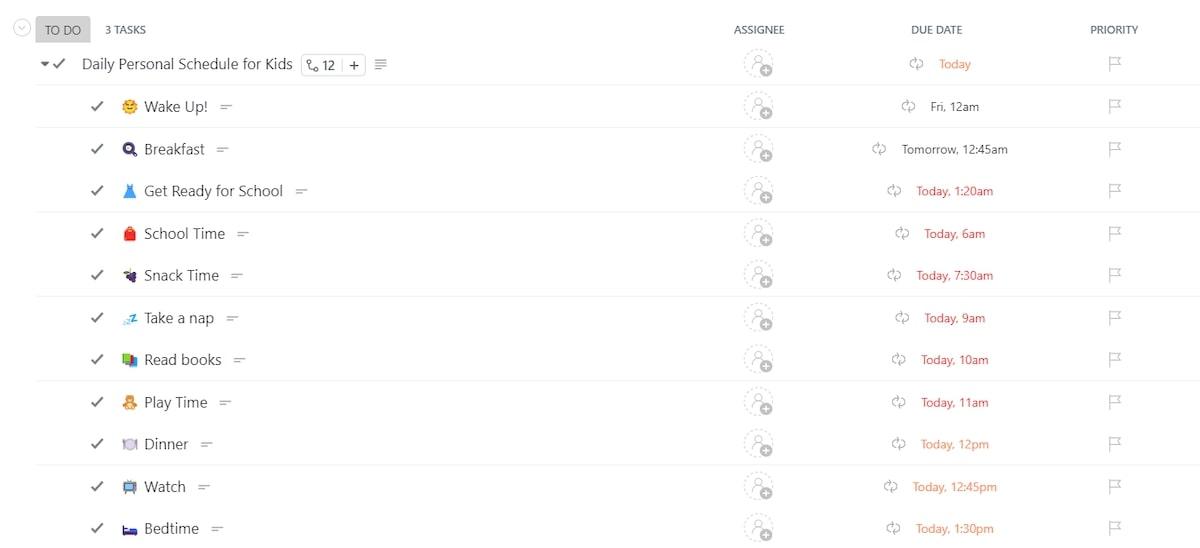Screenshot of a scheduling application displayed on a white background. The top portion of the screen features a gray banner with "TODO" in black letters on the left and "3TASK" to the right. Below this, there is a dropdown arrow followed by a gray check mark. In bold gray letters, the main heading reads "DAILY PERSONAL SCHEDULE FOR KIDS," with a button labeled "12+" to its right.

The schedule is detailed with various activities, each accompanied by a gray check mark on the left and icons representing the tasks:
1. A smiley face icon labeled "WAKE UP," followed by the word "NEXT."
2. An icon of a frying pan with an egg labeled "BREAKFAST," followed by "NEXT."
3. A blue dress icon labeled "GET READY FOR SCHOOL," followed by "NEXT."
4. An orange square labeled "SCHOOL TIME."
5. A strawberry icon labeled "SNACK TIME."
6. A small blue icon labeled "TAKE A NAP."
7. An open book icon labeled "READ BOOKS."
8. An outline of a human body icon labeled "PLAYTIME."
9. A plate on a placemat icon labeled "DINNER."
10. A television icon labeled "WATCH."
11. A bed icon labeled "BEDTIME."

On the far right of the screen, there are three additional columns: "ASSIGNEE," "DUE DATE," and "PRIORITY." The "PRIORITY" column contains checkable flags. The "ASSIGNEE" column includes an option to "ADD A PERSON," and the "DUE DATE" column displays dates and times centrally.